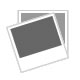This screenshot captures a detailed view of a user's eBay app on their smartphone. The time displayed at the top left corner of the screen is 2:21, while the battery indicator at the top right is halfway full. The eBay page's heading prominently reads "Item," and a shopping cart icon beside it shows that there are eight items currently in the cart. Directly below the heading is an "Add to Watch list" button.

The main part of the page features a clean white background with black text, detailing the specifics of the item for sale. Under the section titled "About this item," the condition is listed as "New with box," and the available quantity is four. The item number is 155742573575, marked with a right-facing arrow beside it.

Further down, additional details describe the brand as "Danger Jones" and type as "Semi-Permanent Hair Dye." The item description from the seller reads: "Danger Jones Ray Gun Neon Yellow semi-permanent hair color, four ounces," also accompanied by a right-facing arrow.

At the bottom of the screen, there's a section labeled "More like this," next to which is a "See All" button.